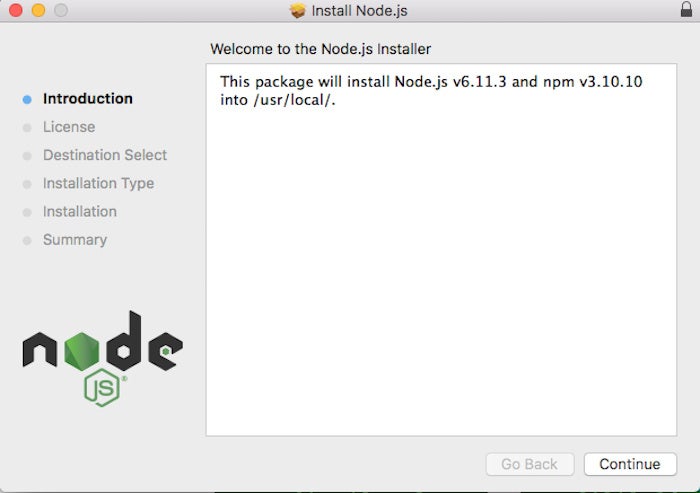The image depicts a webpage specifically designed for installing Node.js. At the very top of the page, there's a menu bar featuring a lock icon, indicating a secure connection. Additionally, the menu bar includes three colored circles whose purpose isn't immediately clear.

Beneath the menu bar is a welcome statement reading, "Welcome to Node.js Installer." The layout of the page is divided into two main sections. On the left side, there are six navigable options that guide the user through different aspects of the Node.js installation process. On the right side, there's a pop-up window that provides real-time feedback on the installation progress.

The pop-up window currently displays a message stating, "This package will install Node.js version 6.11.3 and NPM 13.10.10 into usr/local," detailing the specific versions and target directories for the installation. A "Continue" button is present, which initiates the installation process when clicked. The overall design and functionality of the webpage aim to assist users in easily installing Node.js with clear guidance and progress updates.